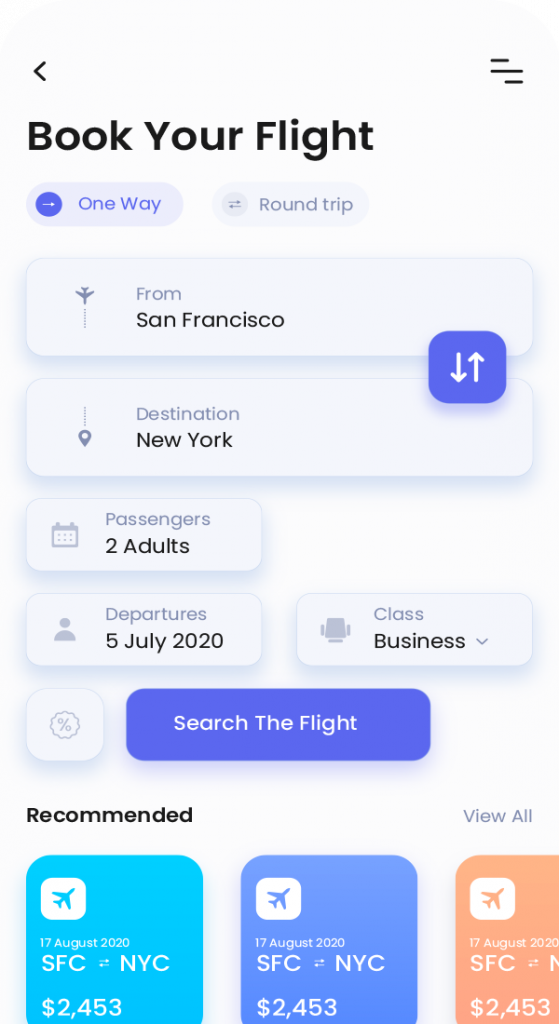The image is a detailed screenshot of a flight booking application interface. At the top, there is a heading that reads "Book Your Flights". Below this, the interface displays several input fields and selections: 

- "One Way" travel from "San Francisco" to "New York".
- "Passengers" are listed as "Two Adults".
- The departure date is specified as "July 5th, 2020".
- The class of travel chosen is "Business".

Under these details, a button labeled "Search This Flight" is prominently displayed. 

Beneath the search button, there is a "Recommended" tab. Within this section, there are three identical cards for flight options. Each card displays:

- The date "August 17th, 2020".
- The route "SFO to NYC".
- The price "$2,453".

The uniformity across all three cards - in terms of date, route, and price - suggests they represent the same flight option repeated thrice within the recommendation tab.